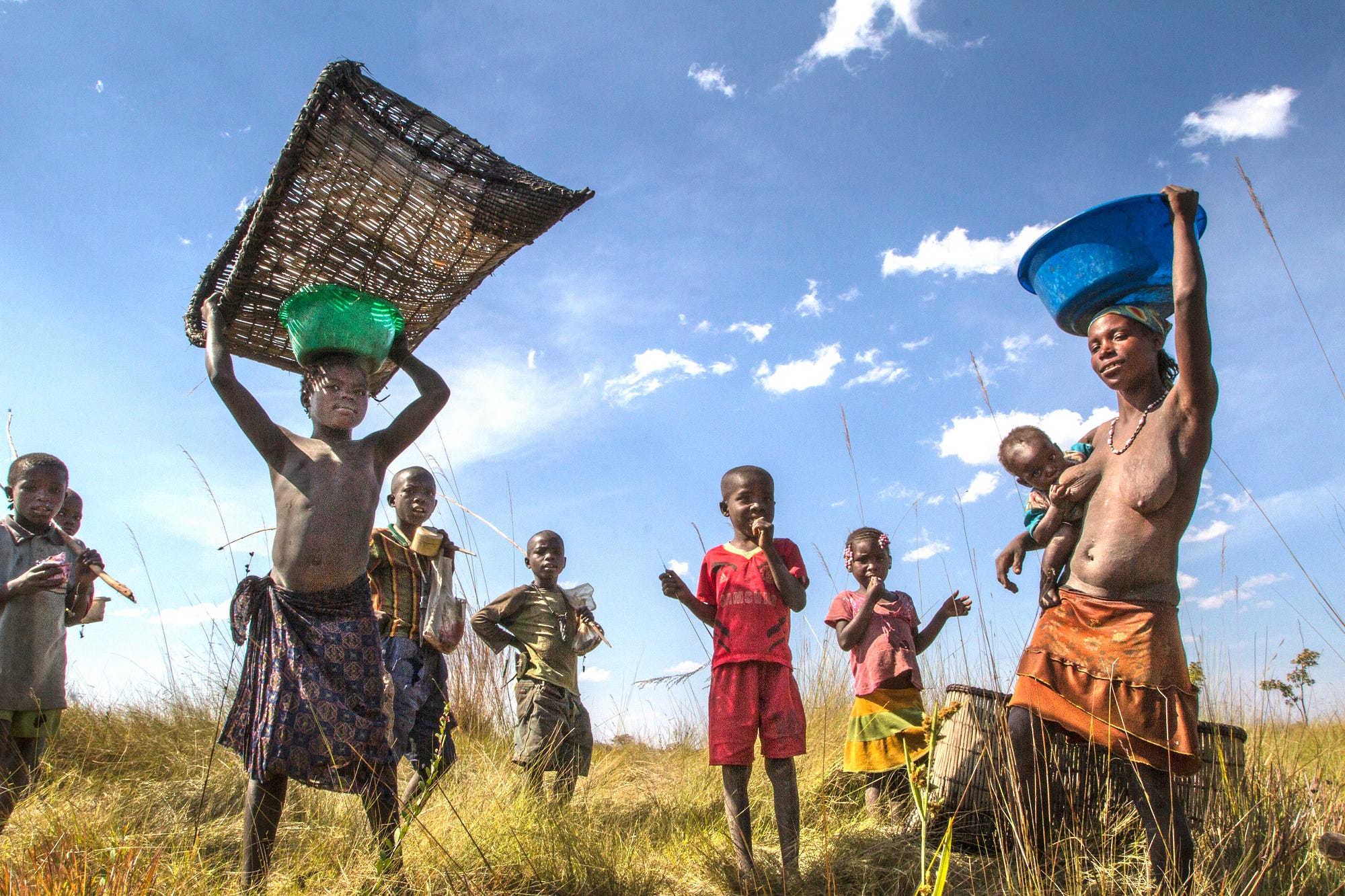In a vibrant grass field with tall, yellowing grasses reaching up to their knees, a group of African children and a woman stand scattered throughout, set against a backdrop of a clear blue sky dotted with white clouds. The children, all with dark skin, exhibit a mix of traditional and minimal attire: some are shirtless with towel-like coverings around their waists, while others wear simple t-shirts. The youngest boys are notable for their bald heads, while the single girl in the group is distinguished by her braids adorned with pink ties.

A young boy stands out with a green bucket on his head, supporting a wooden or bamboo raft-like structure with his small hands. Nearby, a woman, who appears to be the mother, also draws attention; she's bare-chested, breastfeeding a baby, and wearing an orange skirt. Balancing a blue bin on her head, she exudes a commanding presence amongst the children. The scene is a candid glimpse into the everyday lives of this rural community, resonating with the simplicity and resilience of their way of life.